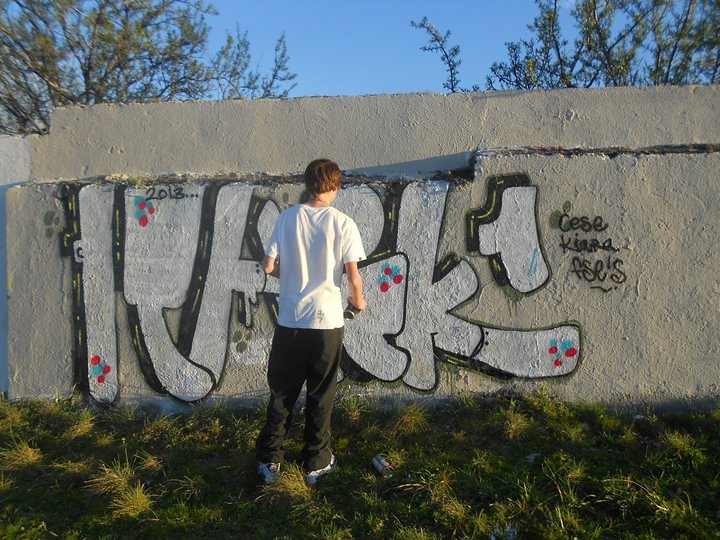A photo captures the scene from behind a young man standing in overgrown grass as he graffiti’s a concrete wall. The background features trees and a cloudless blue sky, while the wall showcases vivid graffiti art. The lettering, predominantly white with black shadowing and adorned with red and blue dots, partly spells out a word with the second letter resembling a "T". The graffiti prominently displays the year "2013". Beneath the artwork, in simpler black writing, is a signature that reads "Sis Kiana FSE!". Scattered in the grass at the wall's base are beer cans, hinting at recent activity.